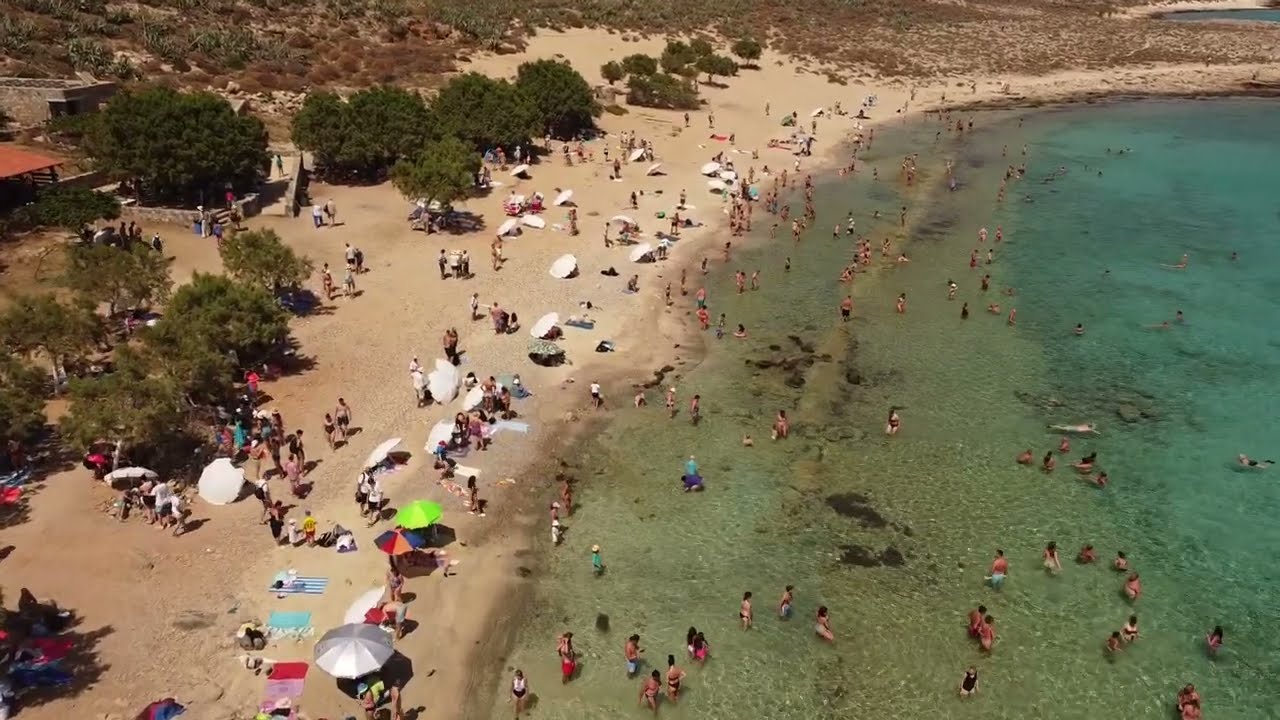The image is an aerial photograph of a bustling beach scene, capturing a lively atmosphere filled with people both in the water and on the sand. The shoreline, characterized by light brown sand, features an array of white and colorful umbrellas along with numerous beach towels. Close to the shore, the sea transitions from a dark green to a bright turquoise as it stretches out into deeper waters. The beach is crowded with individuals enjoying the sun, frolicking, and sunbathing. To the left side of the image, there are lush green trees providing a scenic backdrop, interspersed with rocky hillsides and patches of desert-like landscape with small green bushes. In the far left corner, a structure with an orange roof peeks out from behind the trees, adding an architectural element to the natural beauty of the scene.